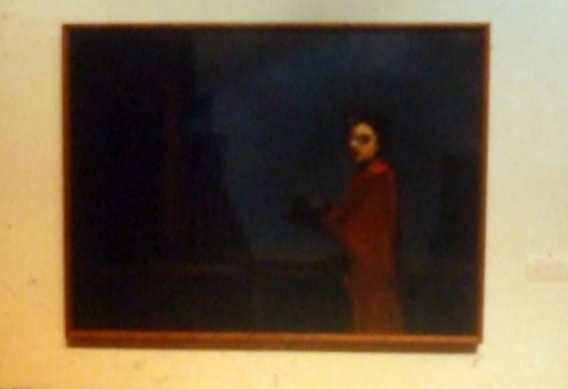The image is a blurry, somewhat dark painting with a square or rectangular shape. The painting itself is predominantly black, bordered by a brown frame. Though the details are difficult to discern, it features a somewhat indistinct figure of a person. The figure appears to be facing forward, and the contours suggest a woman as the subject. She is draped in a long, reddish-brown garment. Her skin tone is medium, neither very dark nor very light. The painting is mounted on a wall with an off-white, yellowish hue.